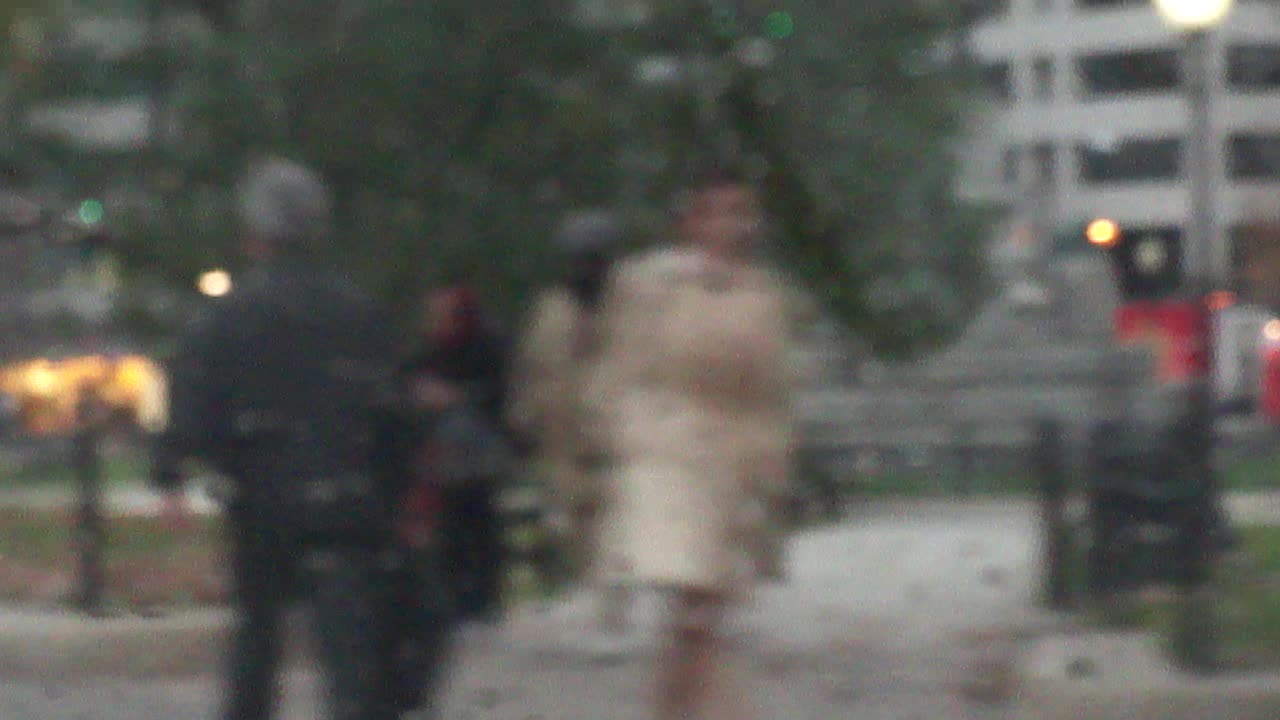In this blurry and distorted photograph, multiple individuals are visible, though details are obscured. At the center, a female figure stands out, possibly dressed in a tan dress or a long tan jacket. To her left, the back of another person—potentially a male—wearing what might be a black police uniform can be seen, though the image’s clarity makes it difficult to confirm. Additional indistinct figures are present in the background. Surrounding them is a verdant scene with a tree and green foliage, suggesting they are walking along a park path adorned with black railings. In the far-right background, a parking garage is visible, accompanied by a light pole in front of it.